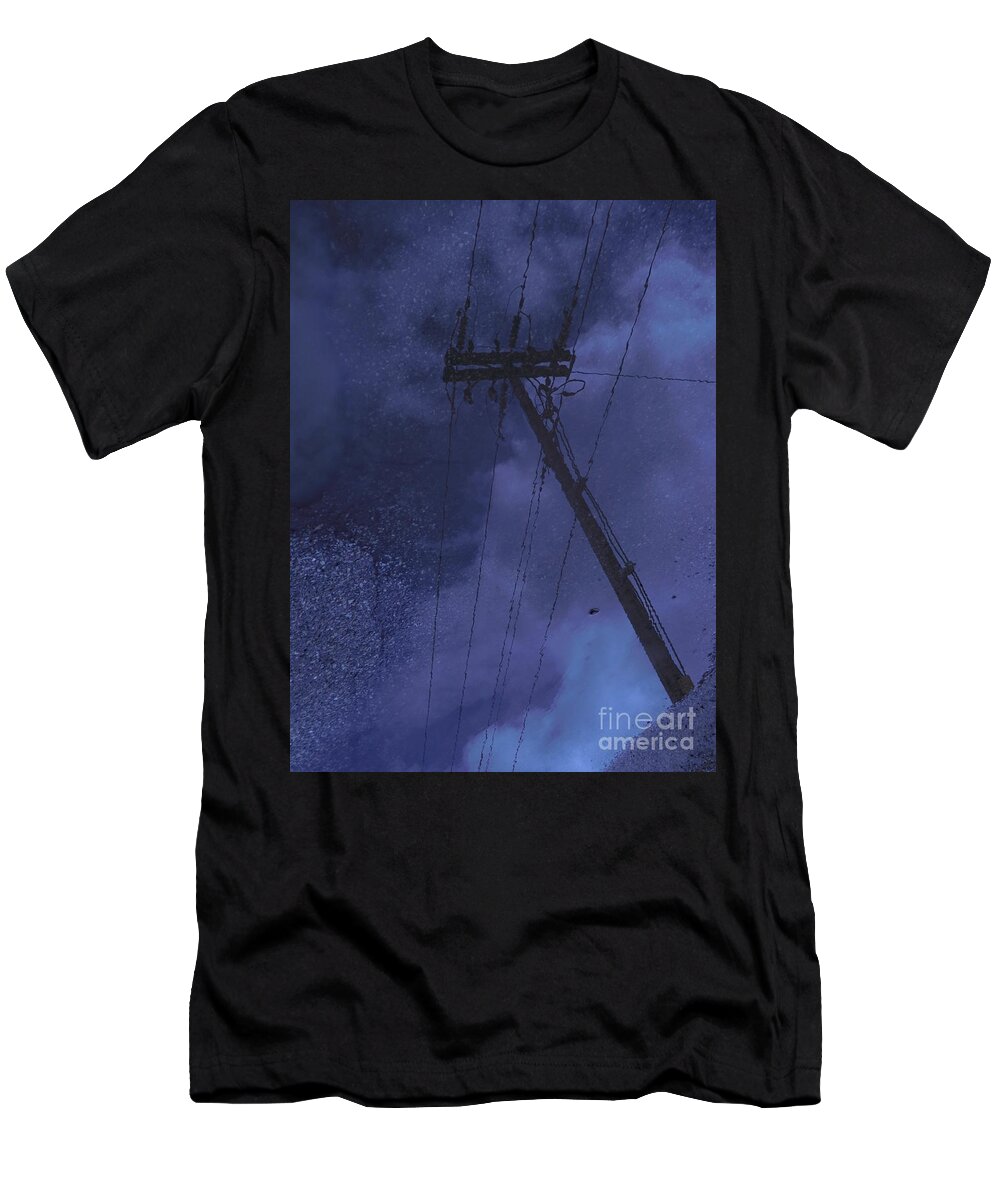This photograph features a black t-shirt adorned with a large, predominantly blue rectangular artwork on the chest. The artwork depicts a bottom-up view of a telephone pole with electrical wires extending into a sky that is composed of blotchy hues of blue and white, adding a moody and somewhat abstract feel. In the bottom right corner of the printed artwork, there is a watermark in white font that reads "Fine Art America." The image of the t-shirt is set against a white background, suggesting that the t-shirt might be available for purchase online. It's worth noting that the artwork appears digitally superimposed onto the t-shirt, as the image does not show any fabric ripples and looks flat, implying that this may be a mockup for an online shop.